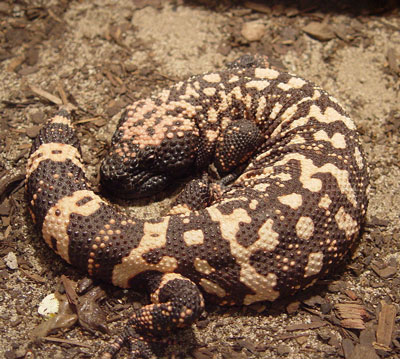The image features a small, curled lizard resting on a brown, fine-grained soil that resembles a mixture of dirt, wood chips, and fine rocks. The lizard is coiled almost completely with its head near its tail, making it look compact. It displays a brown and beige pattern akin to a giraffe's, with a bumpy, scaly texture for camouflage. The lizard's fine patterns render its eyes and nose almost indistinguishable. One leg extends slightly toward the camera. The scene suggests tranquility, potentially indicating the lizard is asleep. The overall environment and the lizard’s camouflage coloration contribute to the serene, naturalistic setting portrayed in the image.